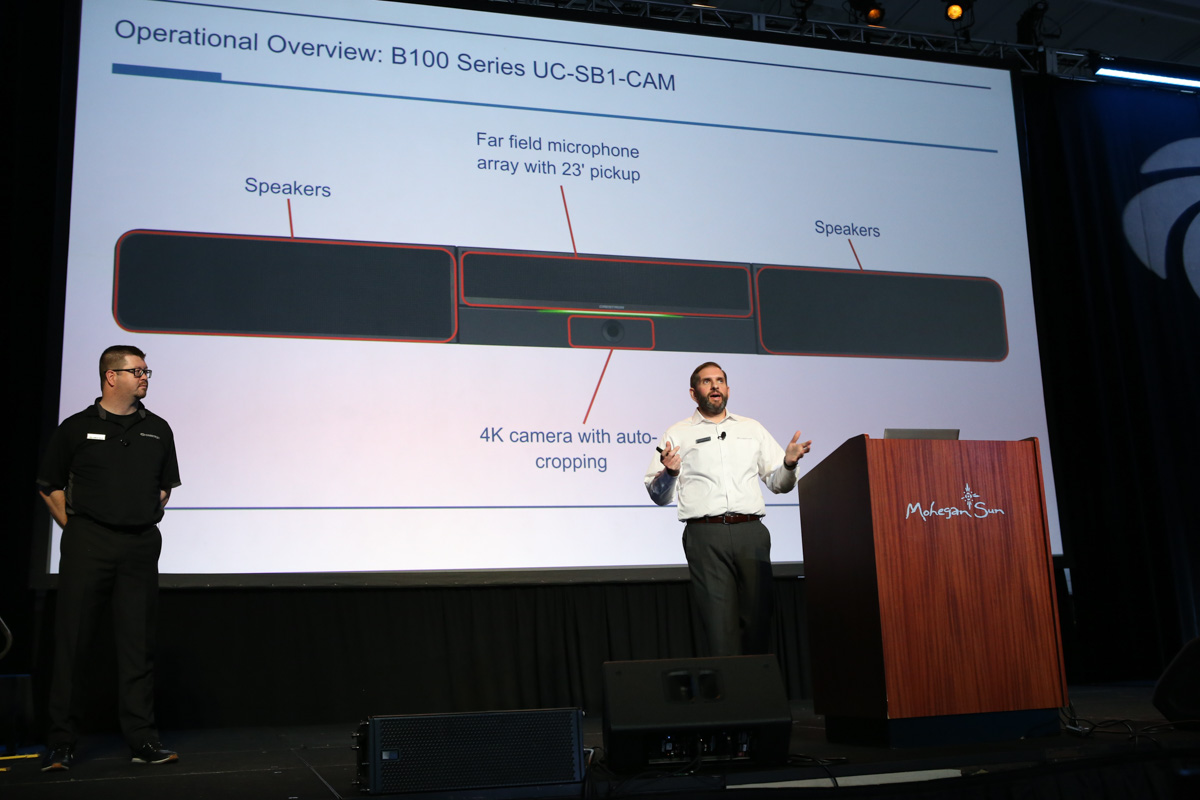The image captures a dynamic scene at a technology conference where a white male presenter with dark hair, a thick beard, and mustache stands on stage giving a speech. Dressed in a white button-down collared shirt and black pants, he is positioned behind a wooden podium that reads "Mohegan Sun." A black microphone is clipped to his shirt, and he stands with his hands open, engaging directly with the audience. To his right, on the left side of the image, another white male with dark hair, glasses, and wearing all black attire — including a black polo and black slacks — watches attentively. The man in black has a logo and a name tag on his shirt, though they are difficult to discern. 

Behind them, a large projector screen dominates the background, displaying the text "Operational Overview B100 Series UC-SB1-CAM." The slide includes detailed images and labels of a piece of audio-visual technology. The technology highlighted on the slide features a "Far Field Microphone Array with 23-Inch Pickup," "Speakers," and a "4K Camera with Auto Cropping." The colors in the setting include mahogany, black, white, red, yellow, green, blue, grey, beige, and tan. Both the podium and stage are situated at the bottom of the setup, grounding the scene of what is clearly a detailed product presentation.